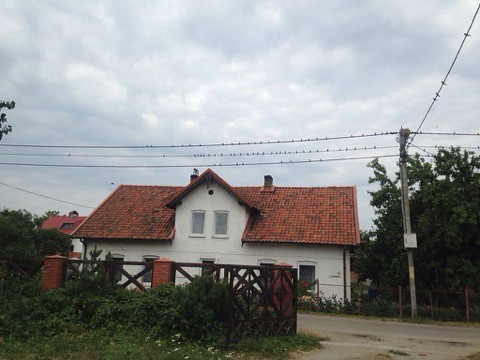The photograph depicts a charming, older white house with a triangular section of the second floor peaking in the middle, covered by a red, brick-patterned roof. The house is adorned with several windows and is set off by itself, suggesting a secluded yet not entirely rural location. In front of the house, there is a black fence made of metal with brick and mortar posts, flanked by green bushes and some white flowers. The scene is accentuated by a main paved road lying between the fence and the house. To the right of the house, a large, lush green tree stands prominently.

Above, numerous power lines stretch across the overcast, cloudy sky, with a power pole positioned to the right of the house. The power lines hold dozens of small birds perched upon them. The sky, densely covered with dark clouds, conveys an impending sense of rain, creating a gloomy yet serene atmosphere. The overall setting appears quaint and picturesque, possibly evocative of a European countryside home.